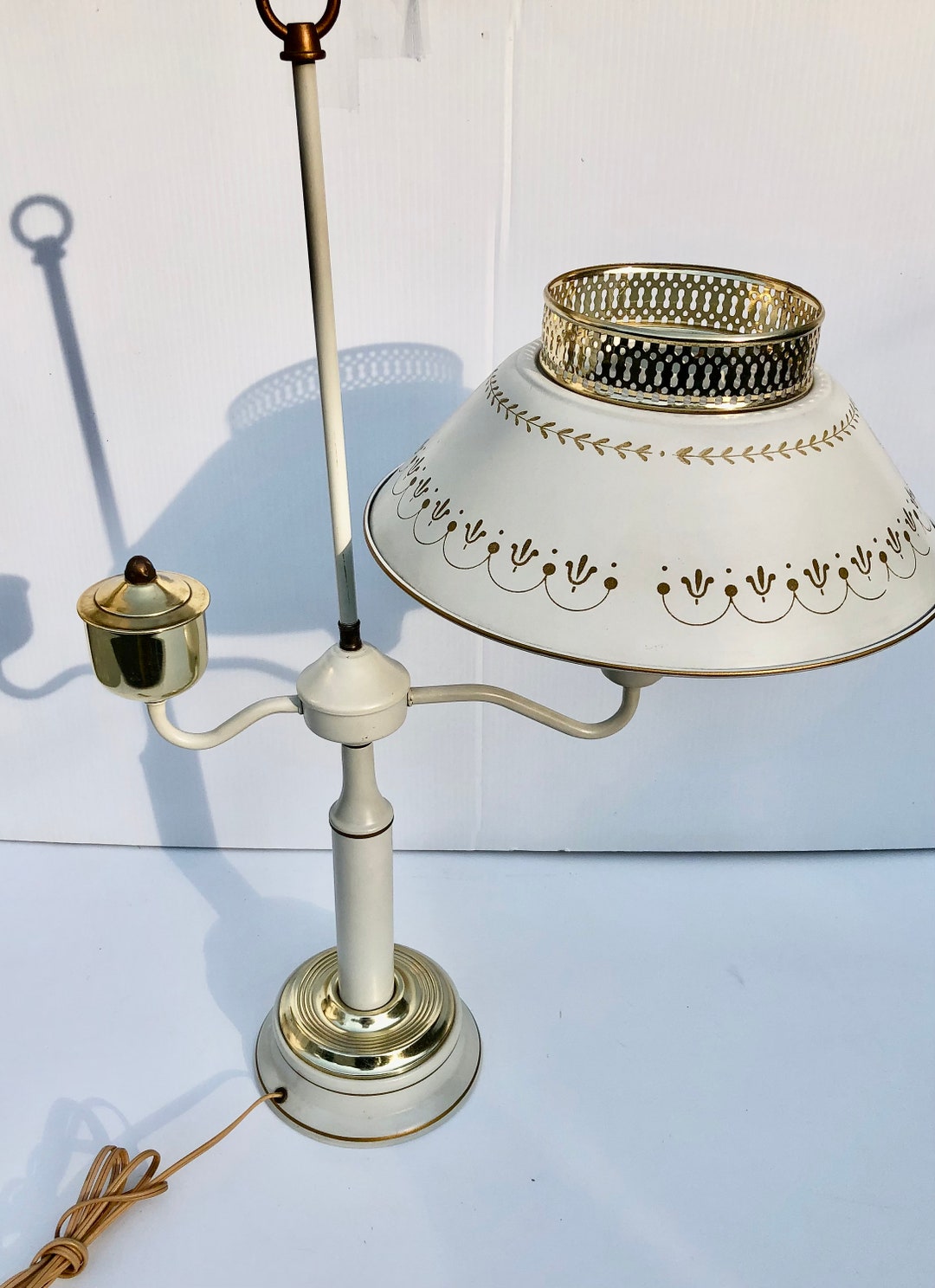This color photograph depicts a vintage living room lamp set against a backdrop of a white wall and positioned on a white surface. The lamp features a long, central pole with two perpendicular arms extending from it; the left arm holds a pot-like object while the right arm supports the light fixture. The light fixture is adorned with an opaque, eggshell white lampshade that bears golden wavy lines and a floral design along its rim. The lamp is marked by gold or bronze metallic accents throughout, including a gold circular area at the top of the shade and a golden metallic base. The base of the lamp has an orange-brown electrical cord that is bundled and trails off the edge of the photograph. The lamp casts a subtle shadow against the white wall behind, adding depth to its old-fashioned aesthetic.